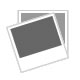This detailed black-and-white advertisement from The Country Gentleman magazine, likely dating back to the 1960s or 70s, showcases a whimsical scene that promotes the Moko Monkey Grip tire patch. The illustration features a man in a tall hat adorned with a stripe that carries the slogan "Save your time, it's money," emphasizing the product as the "greatest time saver ever given to motorists." The man reaches out to receive a can of Moko Monkey Grip from a monkey perched atop the product. The monkey's tail playfully wraps around the can, adding a charming touch to the ad. In the background, a nostalgic rural scene unfolds with a vintage Ford Model T, a farmhouse complete with a silo, a barn, and a tree, evoking a sense of countryside tranquility. The advertisement claims remarkable efficiency, stating that with Moko Monkey Grip, a puncture or blowout can be fixed in just three minutes, ensuring drivers are quickly "on their way." Produced by the Monco Company of America in Oklahoma City, the ad includes a call to action for purchasing the tire patch directly if not available from local dealers, priced at one dollar for a package that guarantees 100 puncture repairs.